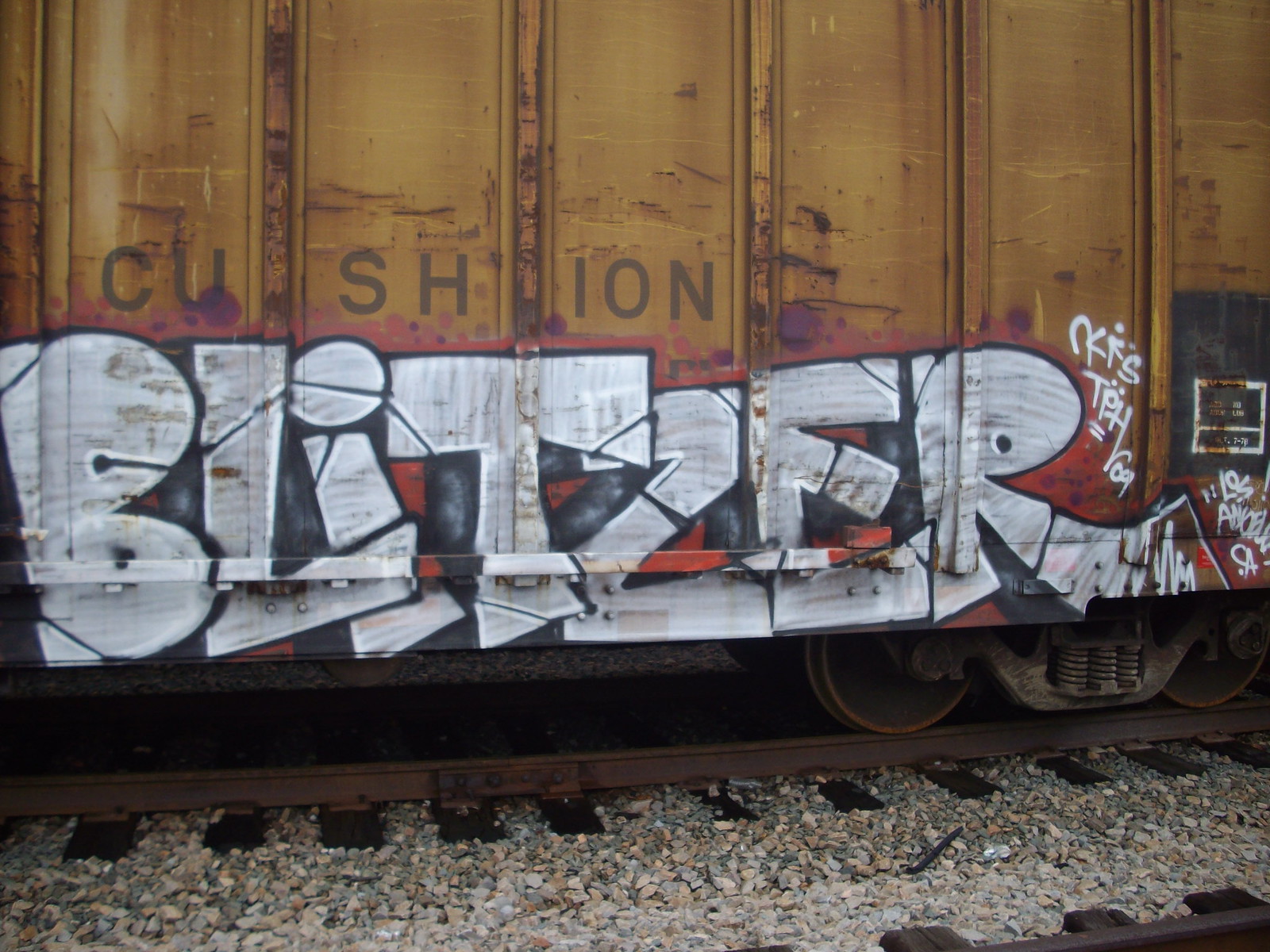This photograph captures a rusty, industrial train car with no windows, painted in a dark yellow-orange hue. The train car, parked on a railroad track with a visible portion of the track and its wheels, displays the word "CUSHION" in dark gray letters across different sections: "CU," "SH," and "ION." Below this text is a prominent piece of graffiti art. The graffiti spells out "Blitzer" in large, bold, balloon-styled letters, painted in a whitish light gray color and accented with red highlights against a black, red, and pink background. There are also traces of less artistic tagging visible on the right side of the car.